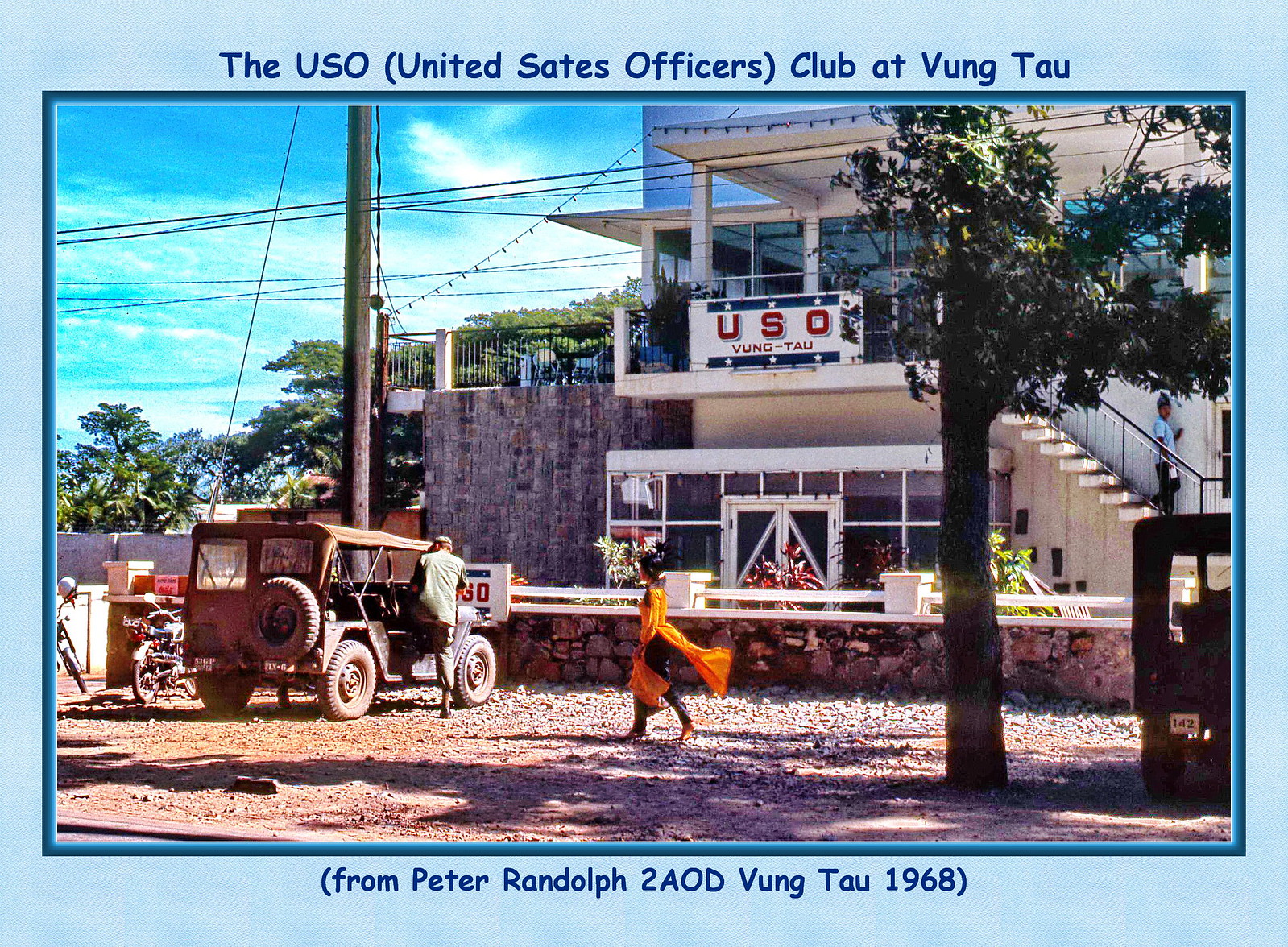This is a detailed color photograph from 1968, featuring a scene captured at the United States Officers Club (USO) located in Vung Tau, Vietnam, during the Vietnam War. The photograph, which seems to resemble a postcard, is mounted on a light blue border. Text across the top reads "USO (United States Officers) Club at Vung Tau," and the bottom text references "from Peter Randolph to AOD Vung Tau, 1968."

In the image, a contemporary-looking building prominently displays a sign that reads "USO" on its second-floor balcony, accessible by stairs on the right. The area surrounding the building is dusty and gravelly, characteristic of the dry environment. 

In the foreground, a military jeep is parked, with a soldier stepping into the passenger side. Adding a sense of motion and liveliness to the scene, a woman in an orange dress—reminiscent of the vibrant hue often associated with Buddhist monks—is seen walking in front of the building, her dress flowing in the breeze. The background showcases a clear blue sky with scattered trees, completing this vivid portrayal of a place where officers would gather during the war.